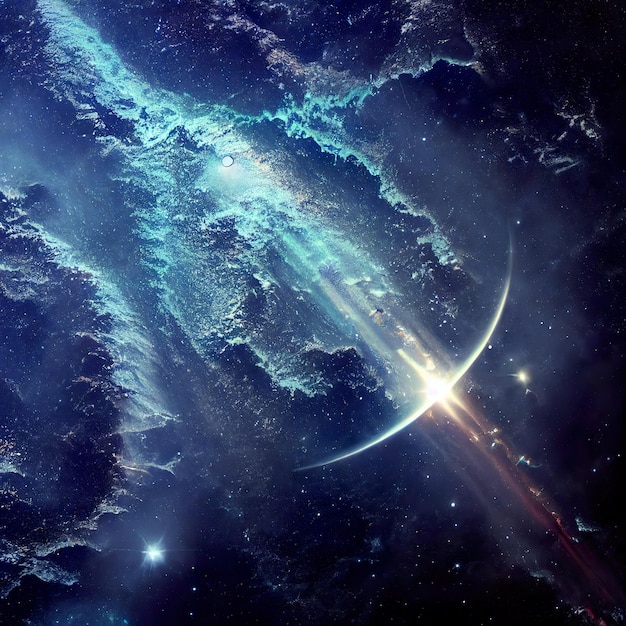This rendered image presents a stunning and intricate scene that blends the ethereal beauty of outer space with the enigmatic qualities of a nighttime sky. The predominant colors are deep blues and purples, enriched by vibrant turquoise hues and accented by streaks of red and yellow light. The backdrop, a dark black and blue sky speckled with bright white stars, features clusters of gaseous turquoise formations. Central to the image is a radiant arc of white light, with a red and yellow streak extending from it. Some interpretations suggest additional elements, such as a meteor illuminating the sky, or the possibility of the moon making an appearance as a sliver of light. Other parts of the image bring to mind an ocean scene with high waves, flooded roads, and car headlights, adding to the overall sense of mystery and depth. This juxtaposition of celestial and terrestrial impressions makes for a truly captivating and evocative visual experience.